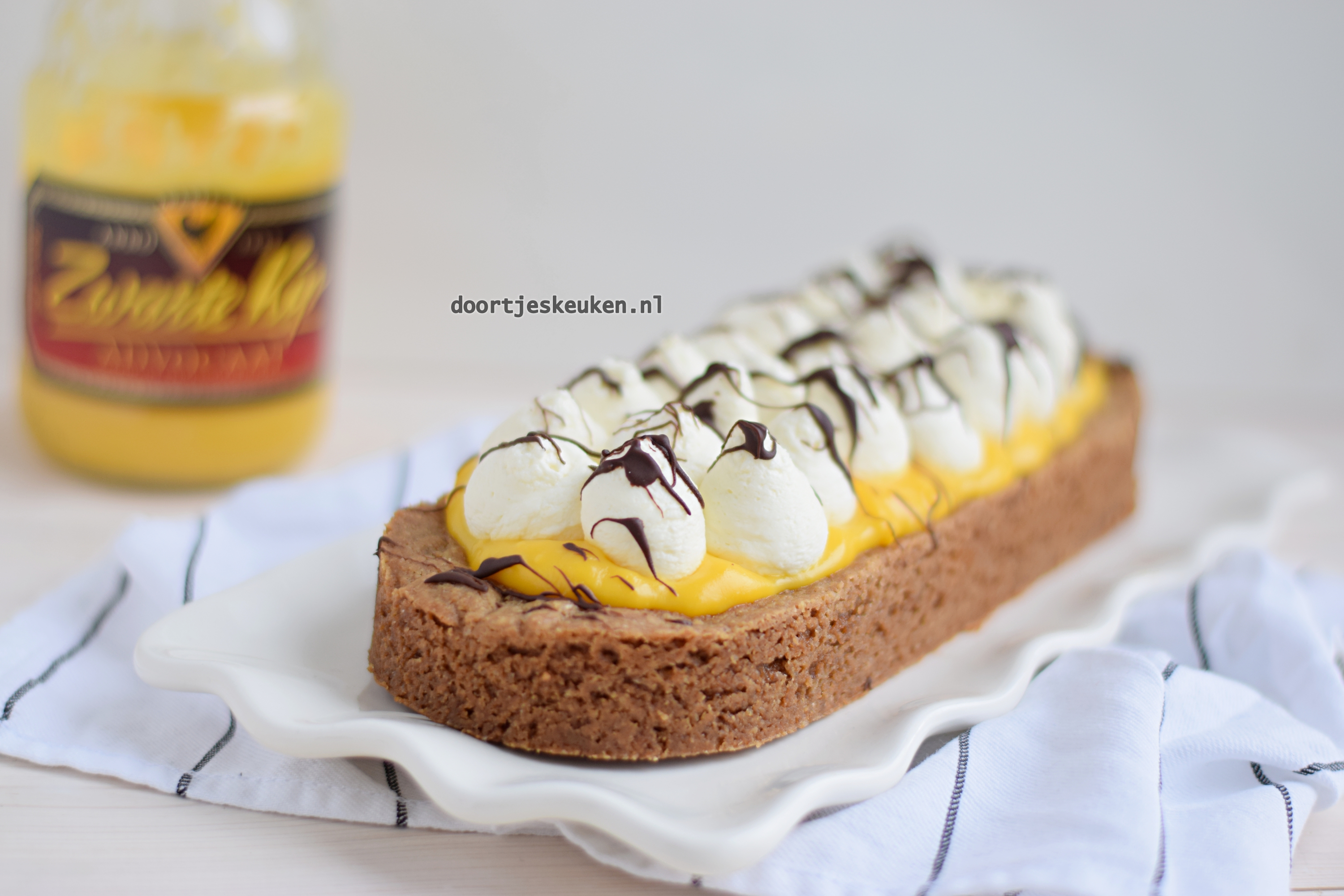The image features a close-up of an elegant dessert, positioned horizontally against a slightly blurred gray background. The treat is a long, oval-shaped cake, with a spongy, brown base that suggests it might be made of gingerbread or a similar cake. Atop the base is a layer of yellow cream, possibly mustard in appearance but more likely a rich custard or lemon curd. The yellow cream is artfully topped with numerous small, white dollops of cream, arranged to resemble miniature Hershey's Kisses, creating a visually appealing contrast. The dessert is further embellished with a delicate drizzle of dark chocolate.

The cake is set on a white plate that features artistically wavy edges, adding a touch of sophistication to the presentation. Positioned beneath the plate is a blue napkin adorned with dark blue stripes. To the left of the dessert, a clear jar filled with a yellow substance, likely lemon curd, has a partially legible label that includes the letters "Z-W-A-R-A-K-Y," and it's adorned with yellow lettering on a black and red background, though the details remain slightly blurry. Additionally, a faint gray inscription in the background reads, "Doerr to Jessica.N1," suggesting a personal message or brand. The photograph is taken at an angle, highlighting the intricacies of the dessert and its surrounding elements, and captures a variety of colors including yellow, white, brown, black, red, and blue. The setting is indoors, and the overall style is a professionally-styled food photograph.